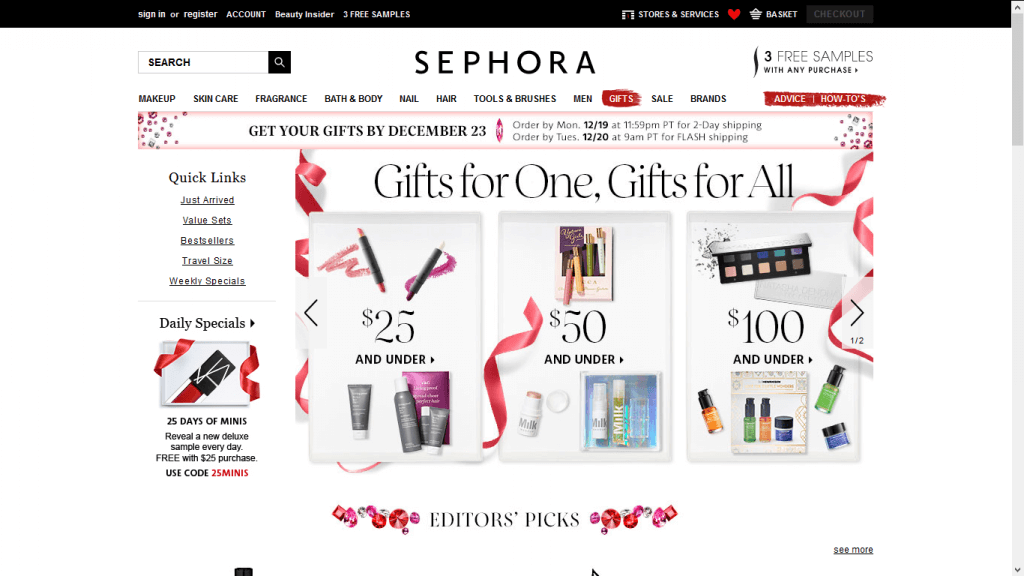The top of the image features a black banner with the following options: "Sign In to Register," "Account," "Beauty Insider," "Three Free Samples," "Stores and Services," and "Basket." Directly beneath it, a search bar labeled "Search Sephora" is visible. The banner also repeats the offer of "Three Free Samples with Any Purchase."

Just below this, a horizontal menu provides categories such as "Makeup," "Skincare," "Fragrance," "Bath and Body," "Nail," "Hair," "Tools and Brushes," "Men," "Gifts," "Sale," "Brands," and "Advice and How-To's."

Further down, an announcement states: "Get your gifts by December 23rd. Order by Monday 12/19 at 11:59 PM PT for Two-Day Shipping. Order by Tuesday 12/20 at 9 AM PT for Flash Shipping."

The main section is divided into three promotional boxes:
1. The left box displays various makeup and skincare products under the heading "25 and Under."
2. The middle box features a selection of other items with the label "50 and Under."
3. The right box presents additional makeup items categorized as "100 and Under."

At the bottom, in grey capital letters, the caption "Edna's Picks" stands out.